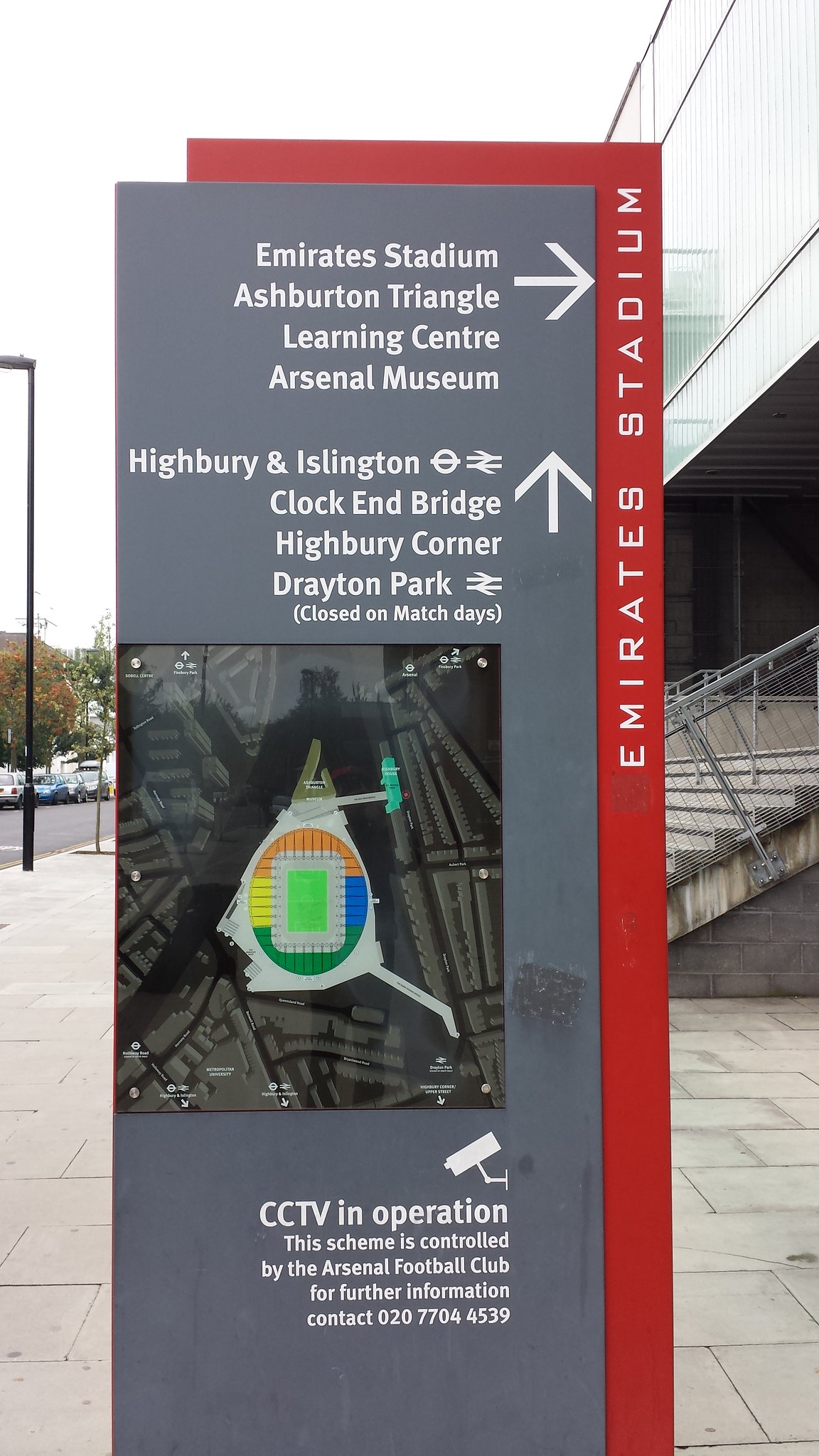The image shows an overcast outdoor setting featuring a tall black lamppost and parked cars lining the street. In the background, you can see some trees and a several-story building with concrete stairs and metal railings. Central to the image is an information board with a red border along the top and the right side, proudly displaying "Emirates Stadium" in vertical writing at the top. The main portion of the board has a gray background with white lettering that gives directions: an arrow pointing right towards "Emirates Stadium, Ashburton Triangle Learning Centre, and Arsenal Museum," and another arrow pointing up towards "Highbury and Islington, Calkin Bridge, Highbury Centre, Drayton Park," with a note that Drayton Park is closed on match days. An aerial view map and a camera icon with "CCTV in operation" are also depicted, the scheme being controlled by the Arsenal Football Club. For more information, there is a contact number provided at the bottom.